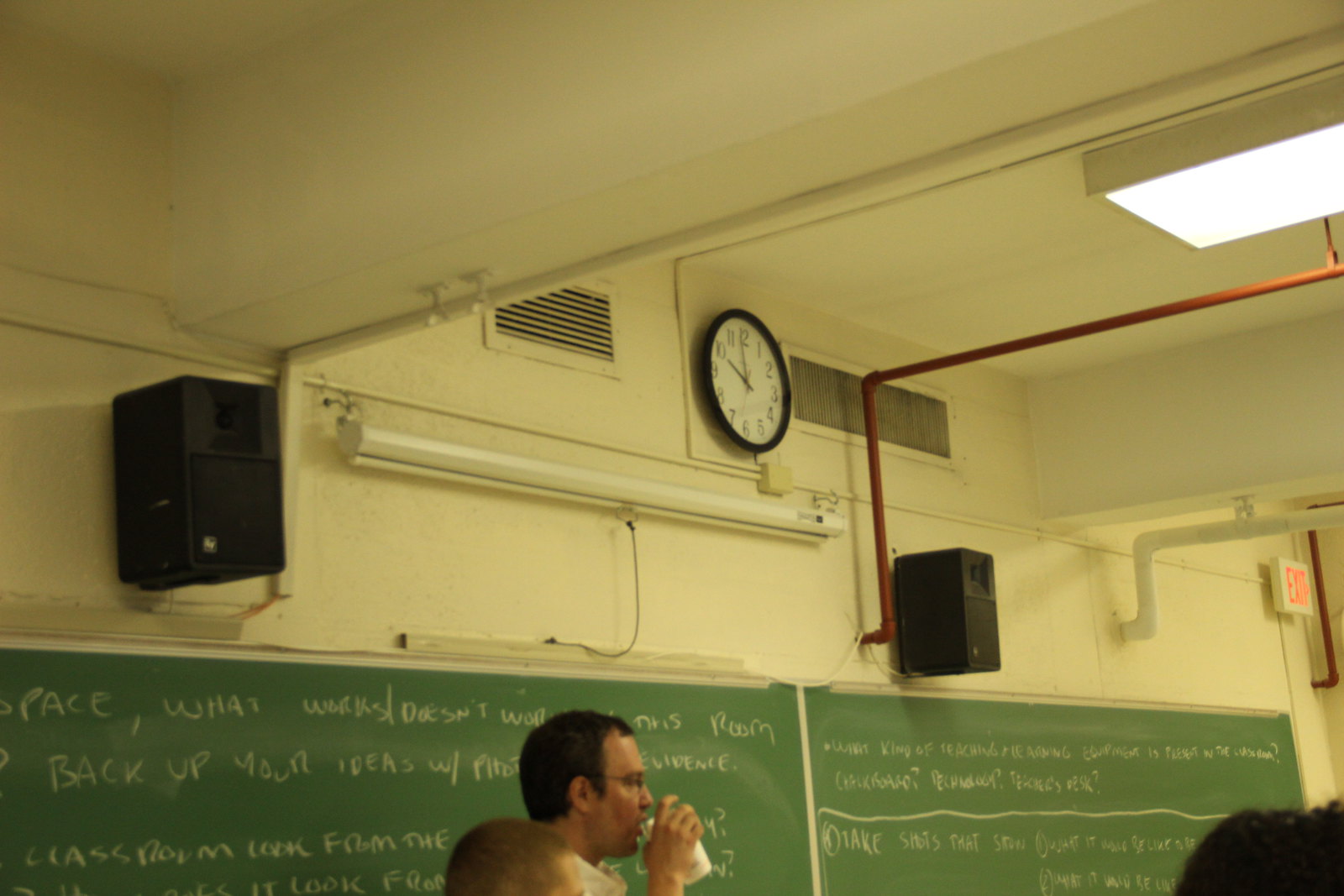The image depicts a high school or college classroom, with the camera angled toward the ceiling and the upper portion of the back wall. At the bottom of the frame, three individuals' heads are visible: one just peeking in from the bottom right with black hair, another centrally located with short, shaved blonde hair visible from the eyebrows up, and a man with short black hair and glasses, captured in profile lifting a white mug to his lips.

The classroom features a greenish-tinged blackboard spanning the bottom quarter of the frame, covered in white chalk writing. Phrases like "back up your ideas with" and "what works/doesn't work" can be partially read, though much of the text is obscured. Above the blackboard is an off-white wall with a horizontal fluorescent light flanked by two black speakers.

A pull-down projector screen, still rolled up in its case, hangs above the blackboard. To the rightmost part of the image, an exit sign is visible. Further up, just below the ceiling, is a clock with a black frame and white face, showing the time to be approximately 10:00 AM. The ceiling is adorned with various metal pipes, some likely for plumbing, along with a sprinkler system and fluorescent lighting, contributing to the room's utilitarian look.